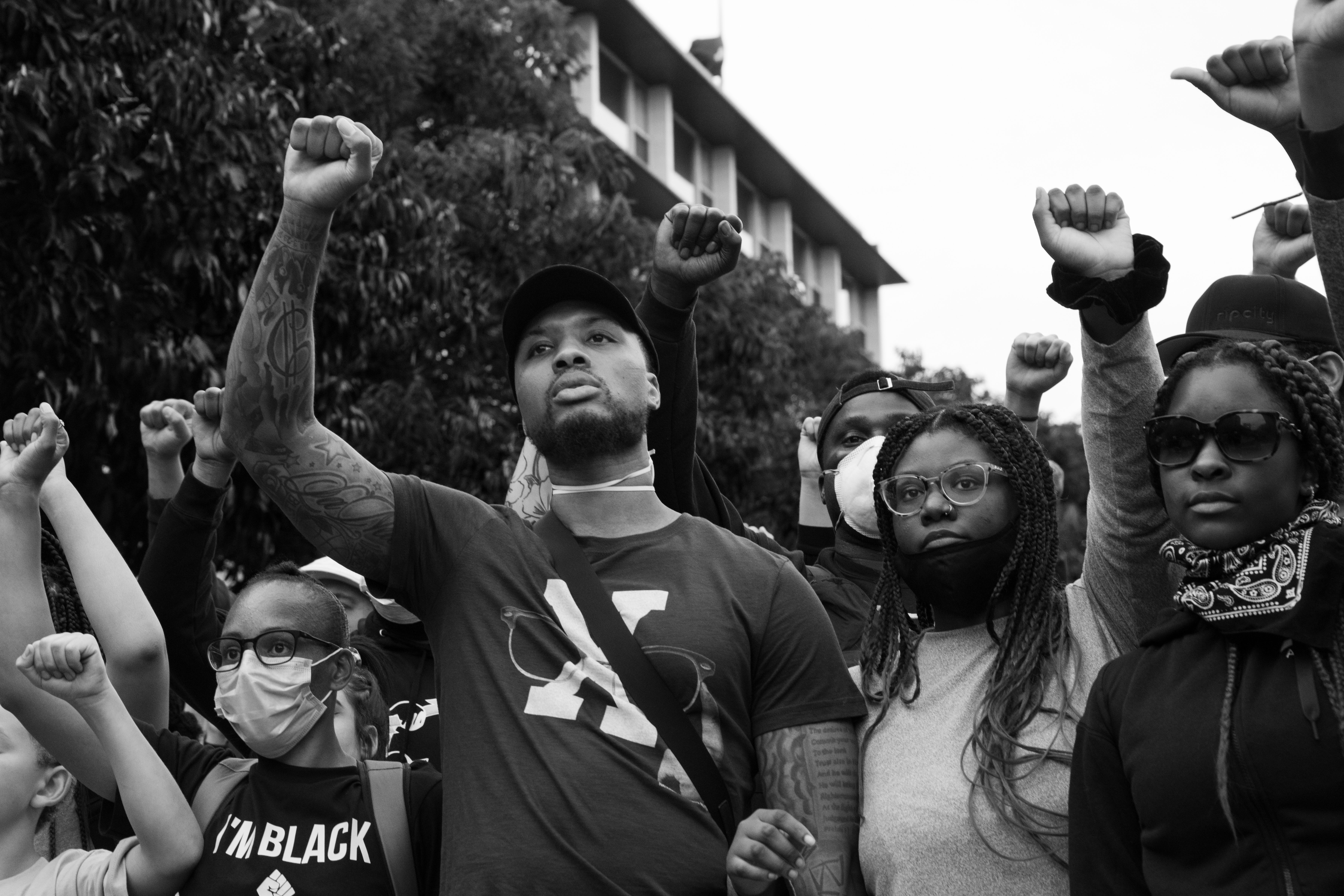In this black and white outdoor image, a diverse group of people is gathered with their fists raised high, symbolizing unity and determination. On the left-hand side, primarily children are seen, each with at least one arm raised. A boy's face is partially visible in the bottom left corner, his fist extended to the right. Next to him, a girl with glasses, her hair tied back, wears a dark-colored shirt with the words "I'm black" written across the chest and has two backpack straps over her shoulders. 

In the middle stands a bearded man wearing a black baseball cap and a black T-shirt with a white 'X' in the center. His right arm, covered in tattoos, is raised in a fist, while his other tattooed arm hangs down. To his right, a woman with long black hair, partially covered in front, wears a white top and glasses. Next to her, another woman in a black jacket, sunglasses, and a bandana, also raises her fist. Between the man and the woman in the jacket, a partially hidden man with a face mask, hat, and dark shirt can be seen.

In the background, there are trees, a white building, and a clear sky, framing the scene of solidarity and shared purpose.